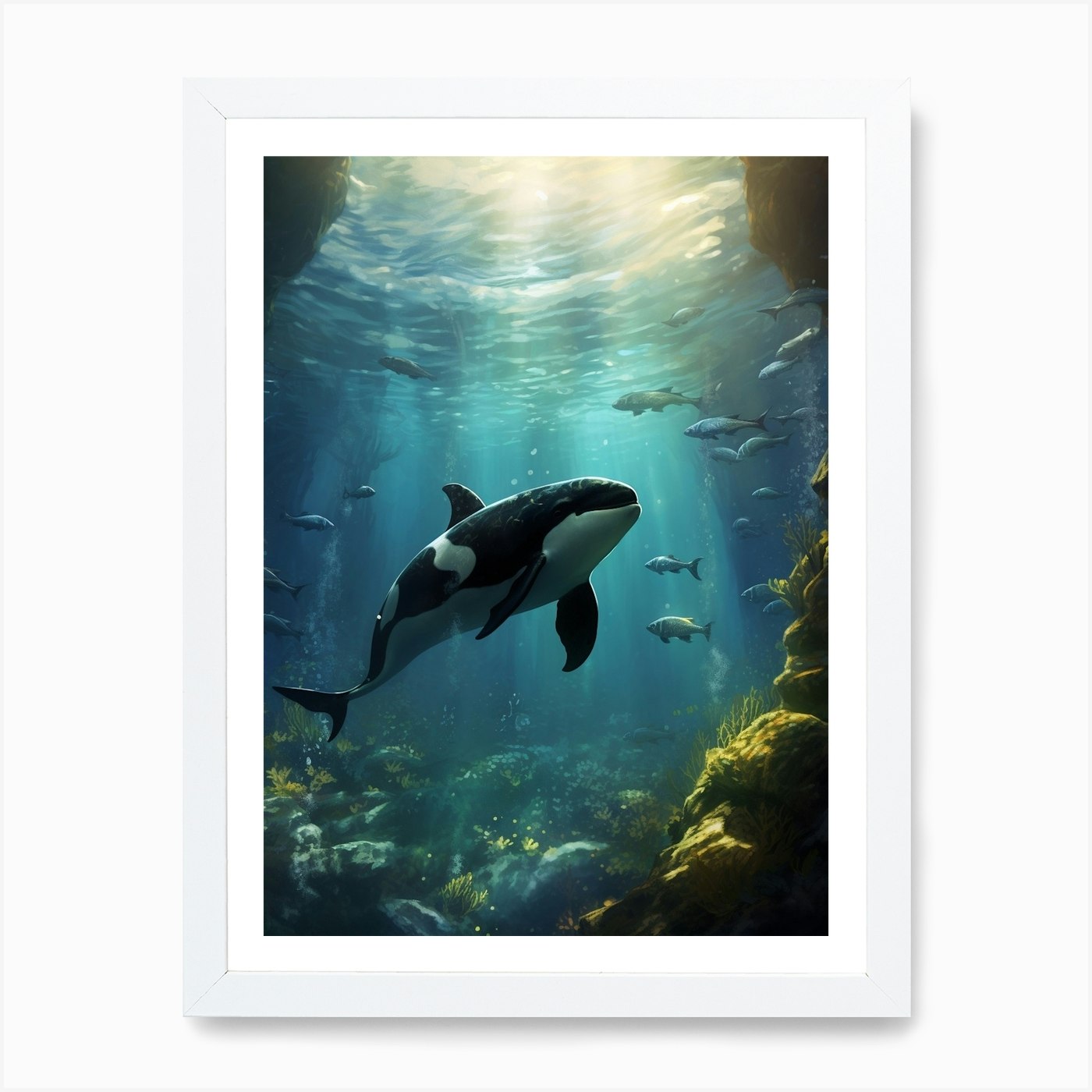This image is an intricate, framed piece of underwater art, captured in a style that appears to be either digitized, watercolor, or oil painting. Dominated by shades of blue depicting the ocean, the central focus is a majestic black and white whale swimming gracefully. The whale's tail fin and other fins are black, while its underbelly and parts of its back are white. Sunlight streams down through the water, creating a serene yet slightly turbulent effect near the surface, depicted in yellow hues. Surrounding the whale, on both the left and right, are various small fish, illustrated in white. The bottom of the scene is rich with marine life, including green and brown algae, coral reefs, rocks, and other detailed plant life such as kelp and seaweed. The attention to detail in the marine environment, combined with the central positioning of the whale, creates a captivating underwater tableau. There is no text within this visually engaging image.